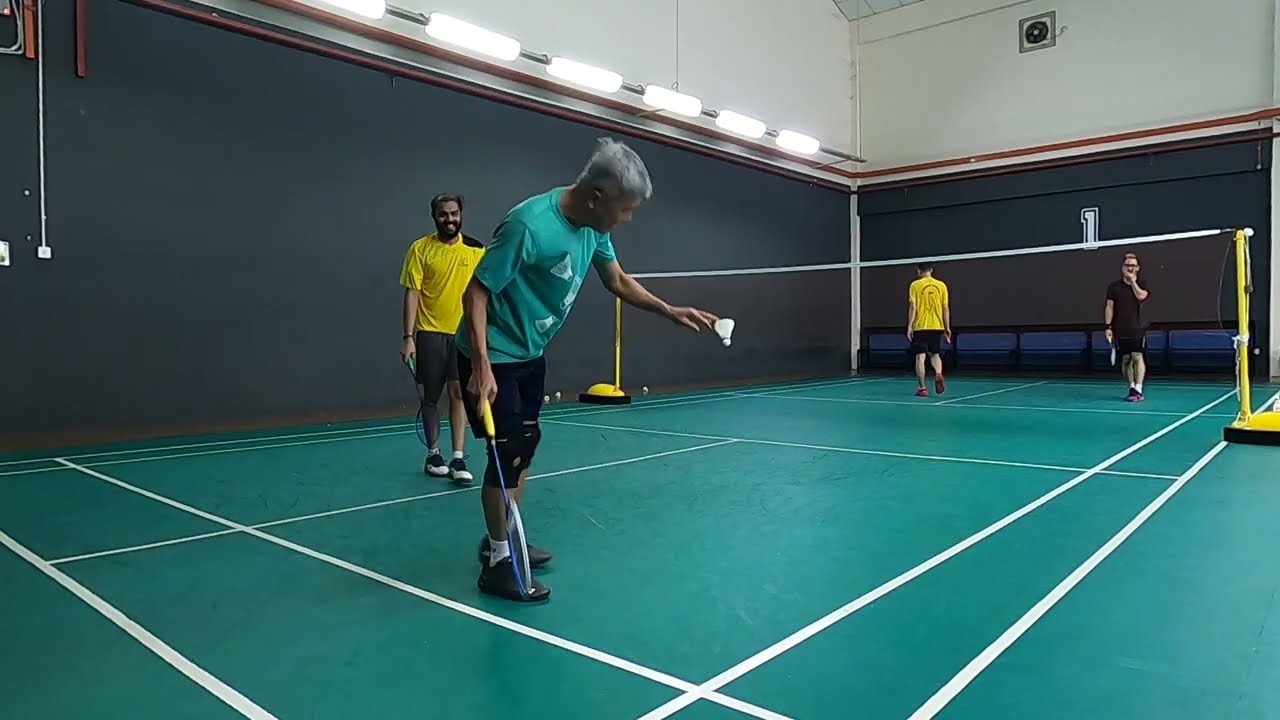The photograph captures an indoor sports facility where four people are engaged in a game of badminton. The court has a greenish, teal flooring, reminiscent of a tennis court. A net, supported by yellow poles on both sides, divides the players into two teams of two. On the closest side to the camera, an older man with gray hair dons a green shirt, black shorts, and knee pads. He is depicted holding a badminton racket and a shuttlecock (birdie). Next to him is a man in a yellow shirt and black shorts. On the opposite side of the net, positioned on the left, is another man wearing a yellow shirt, while to his right stands a man in a black shirt. The facility features white upper walls with black padding at the lower sections, and a series of fluorescent lights that line the left side, some with a bluish hue.